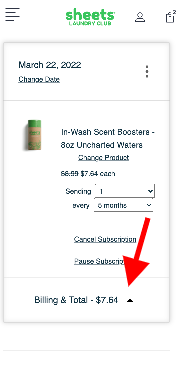The image is a heavily pixelated screenshot, likely taken from a mobile application, with dimensions approximately two and a half times higher than it is wide. 

### Header Section:
- **Top Left:** The top-left corner features a menu icon depicted by three horizontal lines.
- **Center:** At the center, the app's logo is displayed in green text, reading "Sheets." Below it, in smaller text, it states "Laundry Club," although the low resolution makes this text quite difficult to read.
- **Top Right:** Two icons are aligned to the right of the logo.

### Main Content Area:
- **Background:** The main area is enclosed within a light gray rectangle.
- **Date Section:** 
  - **Text on the Left:** The date "March 22nd, 2022" appears in black text on the left side. Below this date is an underlined text, "Change Date."
  - **Icons on the Right:** To the immediate right are three vertical dots.
  - **Divider:** A light gray horizontal line separates this section from the content below.

### Product Information:
- **Left Side:** The left side features a cylinder-shaped image colored tan and green.
- **Text on the Right:** Next to the cylinder, the description in black text reads, "In-Wash Scent Boosters, 8 oz, Uncharted Waters."
  - **Change Product Link:** Below the description, there is another underlined text, "Change Product."
  - **Pricing Information:** Further down, the price "$6.99" is shown crossed out, with the current price listed as "$7.64 each."

### Visual Quality:
- The overall image is very low resolution, making the smaller text and finer details hard to distinguish.

This cleaned-up and detailed caption should give a better understanding of the image's content and layout.